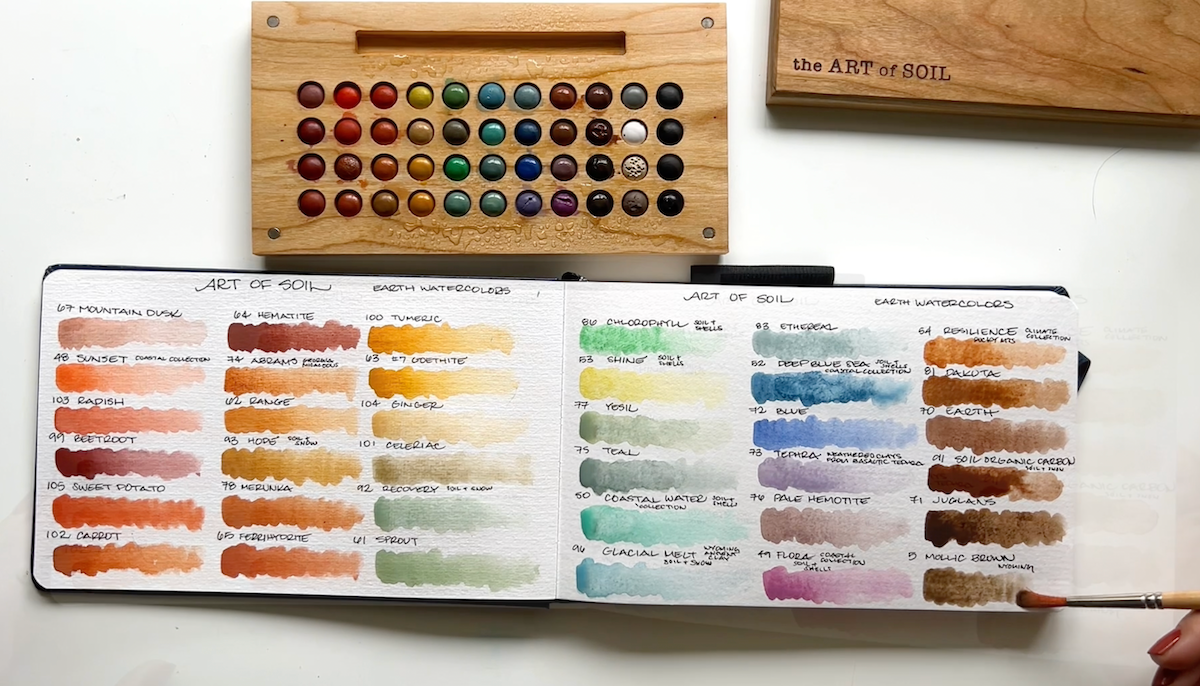This image is a photograph depicting watercolor supplies meticulously arranged against a white background. At the top center of the image, a square piece of light wood holds a grid of small indentations, each containing a marble-sized dot of watercolor paint. These paints are organized in rows following the spectrum of the rainbow, starting from dark red on the left and transitioning through medium red, lighter red, yellow, green, aqua blue, true blue, violet, gray, lighter gray, and black on the right. In the top right corner of this wooden palette, the words "The Art of Soil" are elegantly engraved. Below this wooden board, a rectangular chart displays varying shades of watercolor paint, arranged in columns that range from orange on the left to brown on the right. A woman's finger with a red-painted nail is seen at the bottom right, delicately holding a small paintbrush that touches one of the brown shades on the chart, highlighting the intricate details and vivid colors of these watercolor supplies.